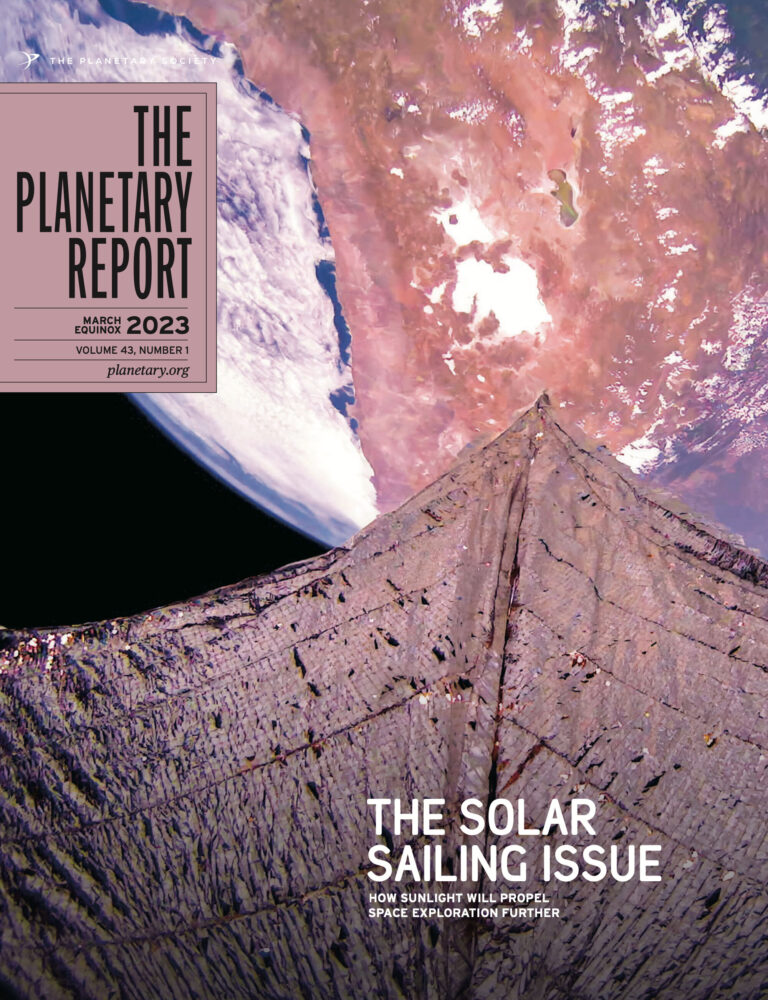The image is likely a cover of a magazine and showcases an advertisement with a striking, intricate design. At the bottom, a tent-like structure is rendered in a fabric-like texture featuring iridescent tan, brown, and metallic colors, lending it a futuristic and ethereal appearance. Prominently displayed in bold, white capital letters at the bottom of the image is the headline: "The Solar Sailing Issue." Beneath this, a compelling subheading reads, "How Sunlight Will Propel Space Exploration Further."

In the upper left corner, a tan square houses the magazine's title in large, black capital letters: "THE PLANETARY REPORT." Directly below this title is the publication detail: "March Equinox 2023." Further down, additional publication information is presented as: "Volume 43, Number 1," followed by the website, "planetary.org."

To the right of these text elements, there is a captivating image depicting Earth as seen from space. This celestial view features various shades of blue, pinkish mauve, and white against a stark black background, providing an immersive glimpse into outer space.